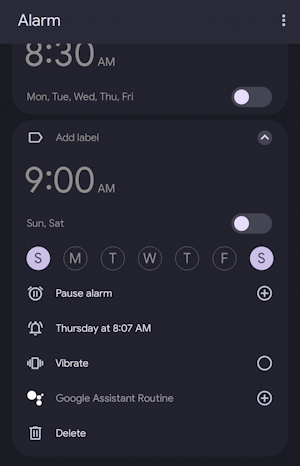The image is a screenshot of a smartphone's alarm clock interface. At the top, there is a black notification bar, and in the bottom right corner of the bar, it reads "Alarm." In the upper right corner, three vertical dots are visible, which, when clicked, provide additional options.

The background of the screen is black. Just below the notification bar, the first alarm is set for "8:30 AM" and is labeled "grapevine." Underneath the time, the days "Monday, Tuesday, Wednesday, Thursday, Friday" are listed, indicating the alarm is set for weekdays. To the right of these days is a toggle switch to activate or deactivate the alarm; it is currently turned off.

Below this section, there is an "Add label" text field accompanied by a label icon to the left. On the far right, there is an upward-pointing arrow allowing the user to collapse this section.

Further down, the second alarm is set for "9:00 AM" and also labeled "grapevine." The days "Sun" and "Sat" (Sunday and Saturday) are displayed underneath, indicating the alarm is set for weekends. Likewise, there is a toggle switch to the right to activate or deactivate this alarm, currently in the off position.

Below the alarms, there are several circular icons representing the days of the week: "S, M, T, W, T, F, S." The circles for "S" (Sunday) and "S" (Saturday) are highlighted with a light purple color, signifying the active days for the weekend alarm.

At the bottom of the screen, there are additional options: "Pause alarm Thursday at 8 or 7 AM," "Vibrate," "Google Assistant routine," and "Delete."

This comprehensive description captures the details and functionalities displayed in the screenshot.